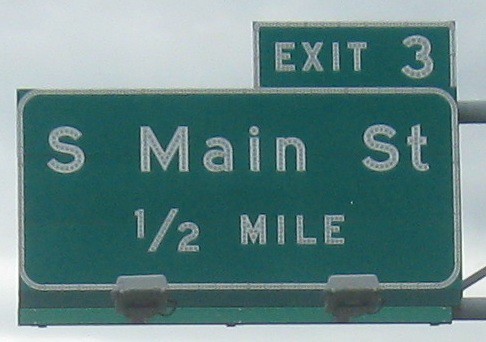The photograph captures a green freeway sign prominently positioned against a partly cloudy, grayish daytime sky. The sign consists of a large rectangular section and a smaller rectangle on the top right. The smaller rectangle in the top right corner displays "Exit 3" in white text. The larger section of the sign reads "South Main Street" in bold white letters, with "½ mile" indicated below in a smaller font. At the bottom edge of the sign, two small lights are visible, likely intended to illuminate the sign for nighttime drivers. The sign is supported by metal poles, which are also faintly visible against the sky in the background. The overall green and white color scheme is characteristic of standard freeway signage, and the image provides a clear representation of what a motorist would typically observe while traveling on the freeway.